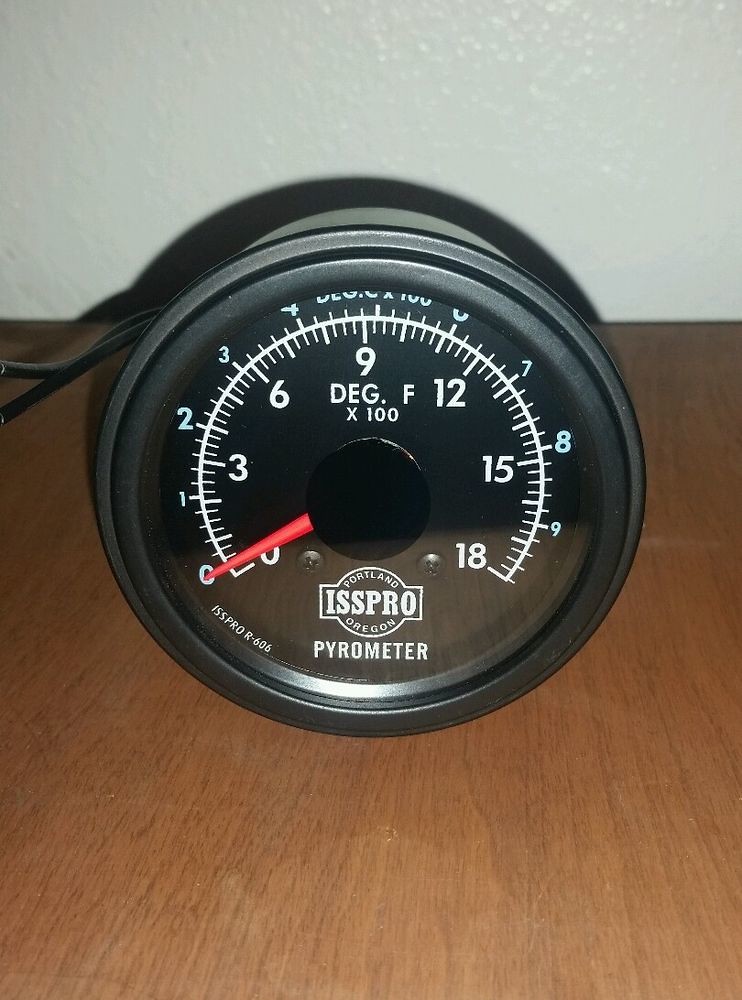This detailed close-up photograph captures a pyrometer, a precision measuring device designed to gauge temperature with high accuracy. The pyrometer, prominently labeled "pyrometer" twice, features a circular face encased in a robust black plastic housing. The face of the device, protected by a clear plexiglass cover, has an inner black dial with two scales: an outer scale ranging from 0 to 9 and an inner scale ranging from 0 to 18, both marked by crisp white numbers. A vivid red needle at the center of the dial points to the readings, similar in style to a thermometer or speedometer. This indoor shot was taken on a wooden table against a backdrop of a plain white wall. Connecting to the bottom of the pyrometer are two thin cables, possibly for power or data transmission. An inscription on the device indicates that it is manufactured by ISPRO in Portland, Oregon.